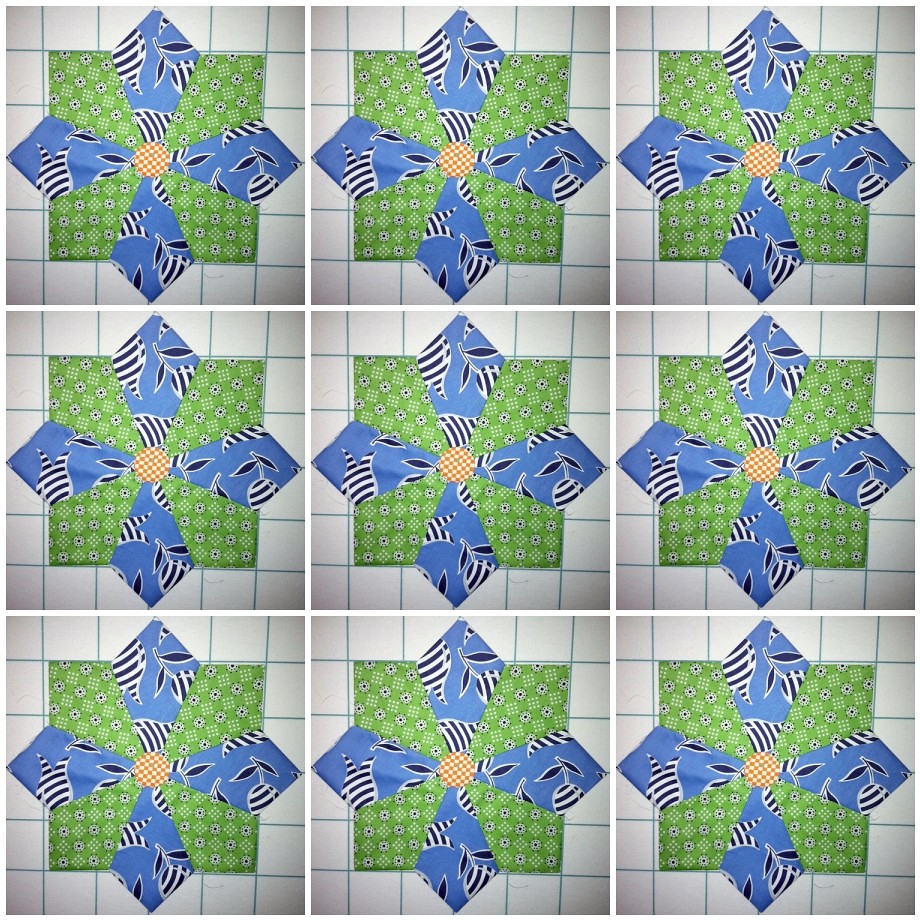This image features a symmetrical arrangement of nine identical squares, each measuring the same size and displayed in a grid of three rows by three columns. Each square showcases a detailed floral design set against a green background. The focal point of each square is a unique flower with four sharp, blue petals adorned with intricate black and white vine and leaf accents. The heart of the flower is a checkered orange and white circular center. Surrounding this central motif, the green background is decorated with white floral elements and small, checkerboard-like patterns. Despite the precise repeating details, the squares appear to be quilting squares rather than tiles, potentially intended for a quilt but laid out merely for display in this image. The harmonious repetition of the design elements across all nine squares creates a cohesive and visually appealing composition.